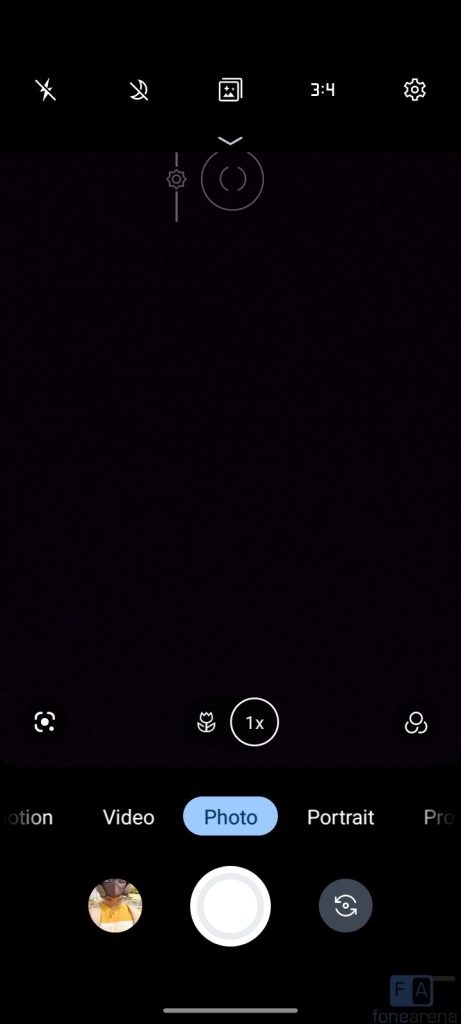The screenshot depicts the interface of a camera application open on a smartphone. The top portion of the screen is entirely black, indicating the camera is either in a dark environment or pointed at an unlit surface. 

At the upper left corner, the flash icon is visible and currently deactivated. Adjacent to it is a crescent moon icon, also turned off, likely representing a night mode setting. The center icon, resembling a camera, indicates the photo capture function. To its right, an icon denoted by a fraction, possibly 3/4, suggests an option to change the image size. The far-right gear icon accesses the full settings menu.

Dominating the lower middle section of the screen is a prominent white circular button for capturing photos. To its right, a rotating arrows icon allows switching between different camera orientations, such as portrait and landscape modes. On the left, a small thumbnail of the last photo taken is visible, though its details are indistinguishable.

Above these, a highlighted blue icon signifies that the app is currently in photo mode. Flanking this photo mode icon are options for video mode on the left and portrait mode on the right, both indicated by their respective icons.

The overall layout and active features suggest that the user is poised to take a photograph but has not adjusted any settings or activated additional features yet.